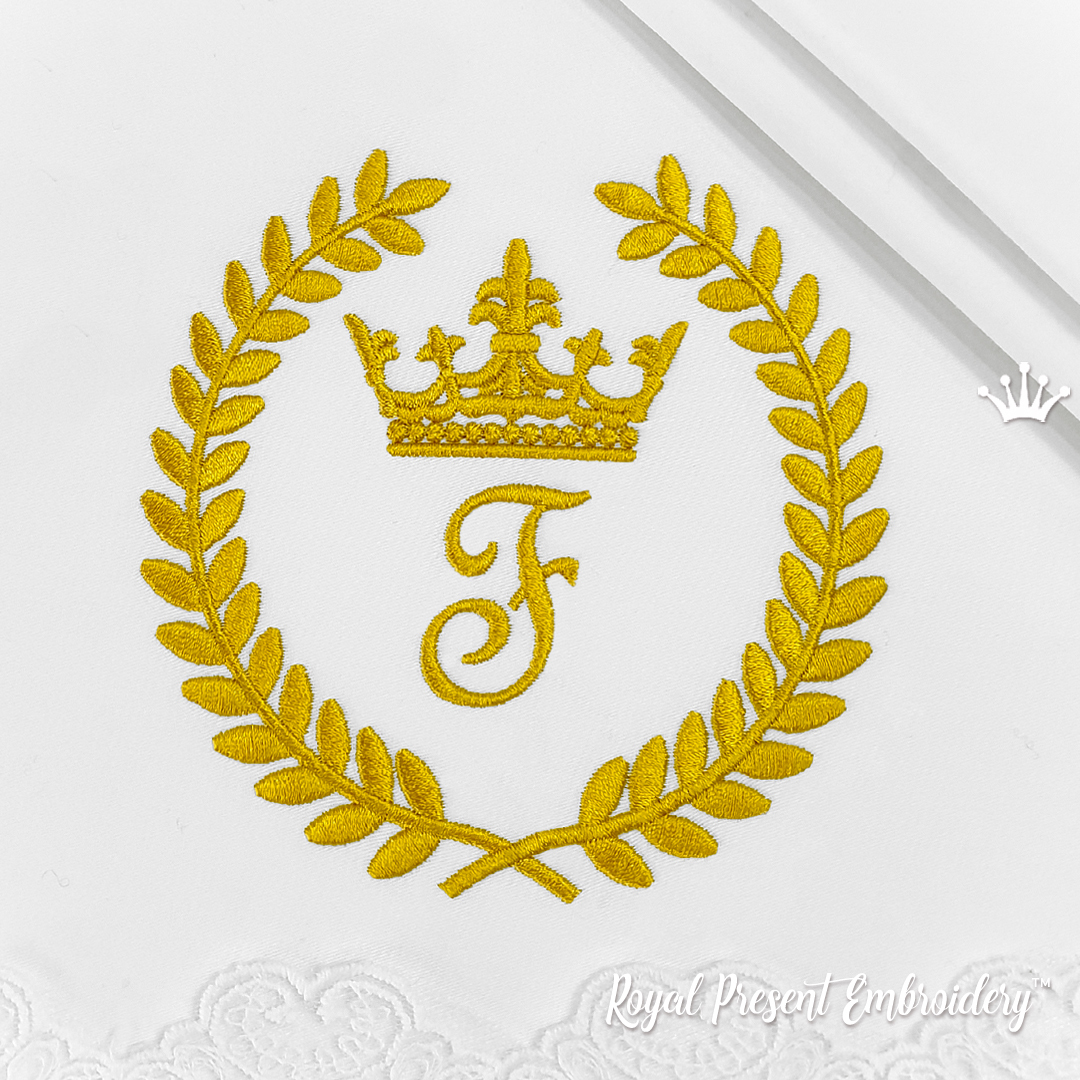The image depicts a detailed close-up of luxurious white cotton or linen fabric, potentially linenware, adorned with intricate golden embroidery. The centerpiece is an opulent crest featuring an ornate, circular monogram with a cursive letter "F" and a regal crown at the top, both embroidered in rich golden thread. Encircling the monogram are two laurel branches or fronds with approximately 20 small leaves on each side, nearly meeting at the top. Below the embroidery, the fabric showcases delicate lace-like ruffles or white-on-white embroidery along its edge, adding an extra touch of elegance.

This image is branded with watermarks from "Royal Present Embroidery," with their trademark text placed at the bottom right and their logo, a small white crown, watermarked higher up. Subtle lines run diagonally in the top right corner of the image, giving it a sophisticated, napkin-like appearance. The entire scene is clearly designed to advertise the high-quality embroidery services offered by Royal Present Embroidery.